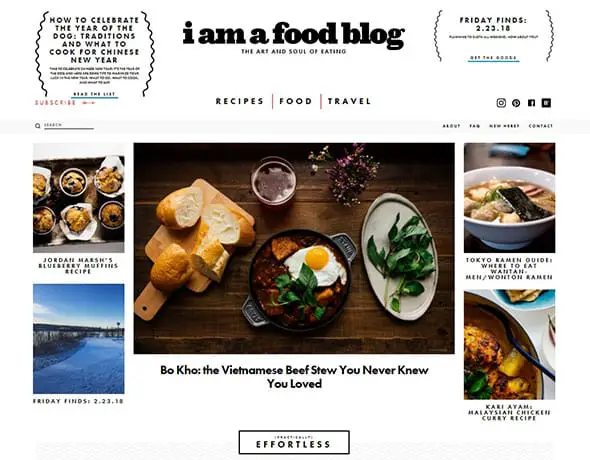**Caption:**
The screenshot features a web page from "I Am a Food Blog," characterized by its monochromatic design with black lettering on a white background. Titled **"How to Celebrate the Year of the Dog: Traditions and What to Cook for Chinese New Year"** (with a hint of humor suggesting "hopefully not dog"), the page centers around an article dated February 23, 2018, titled **"Friday Finds 2-23-18."** Key elements of the page include various sections:

1. **Five Food Images:**
   - **Upper Left**: Jordan Martian's blueberry muffins recipe.
   - **Upper Right**: A steaming bowl of Tokyo ramen.
   - **Center**: A chili bean pot stew with a perfectly poached egg on top, served with a side of bread.
   - **Lower Right**: Malaysian chicken curry.
   - **Lower Center**: An unspecified frozen lake image titled "Friday Finds."

2. **Menu Options**: The top menu offers links to Recipes, Food, and Travel, reinforcing the blog’s diverse content.

3. **Main Article Spotlight**: The primary feature is on "Boko: The Viennese Bistro You Never Knew You Loved."

4. **Footer Element**: At the bottom, a brown square features the word "Effortless," possibly indicating a section or a tagline of the blog.

The page exemplifies the blog's dedication to exploring culinary traditions and recipes, blending a mix of cultures and cooking styles into its content.